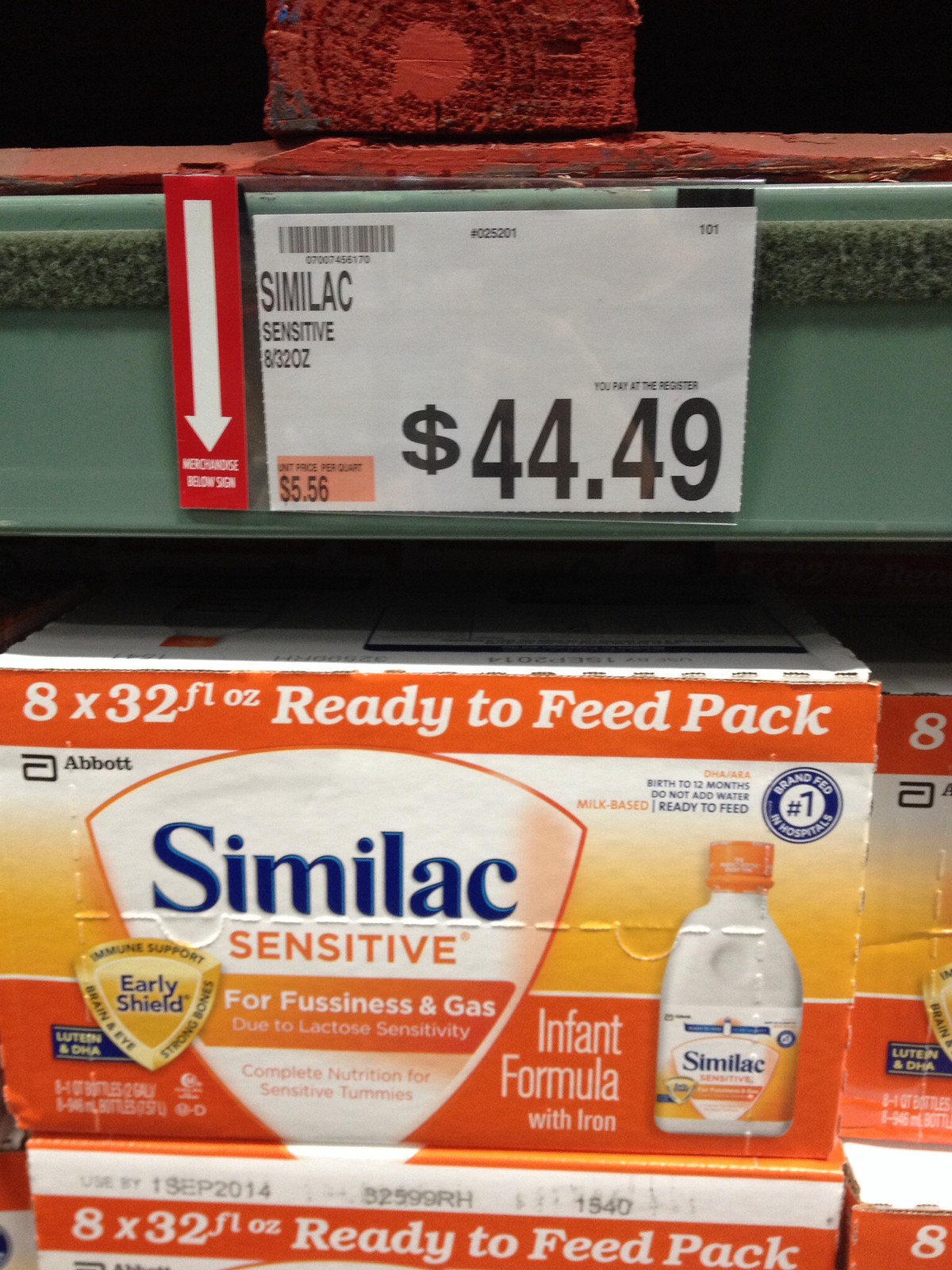This image, taken in a store or pharmacy, showcases a shelf stocked with Similac Sensitive infant formula. Prominently displayed is a large white, orange, and yellow box of the formula. The box features blue and white text detailing "8 by 32 fluid ounce ready-to-feed pack," alongside a picture of one of the individual bottles inside. The text further specifies "Similac Sensitive for fussiness and gas, infant formula with iron." The box is positioned on top of another similar box, flanked by at least two more boxes of the same product. Above the products, attached to a green shelf, is a price tag sign. This sign, featuring a white arrow on a red background pointing down, states "Similac Sensitive, 8/32 ounce" in black text on white. It highlights the price of $44.49 and notes a savings of $5.56. Additional small text, logos, and a barcode are visible but not entirely readable. The overall setting and detailed labeling make it clear this is a section of a retail environment where baby formula is sold, specifically targeting parents with infants experiencing fussiness and gas due to lactose sensitivity.